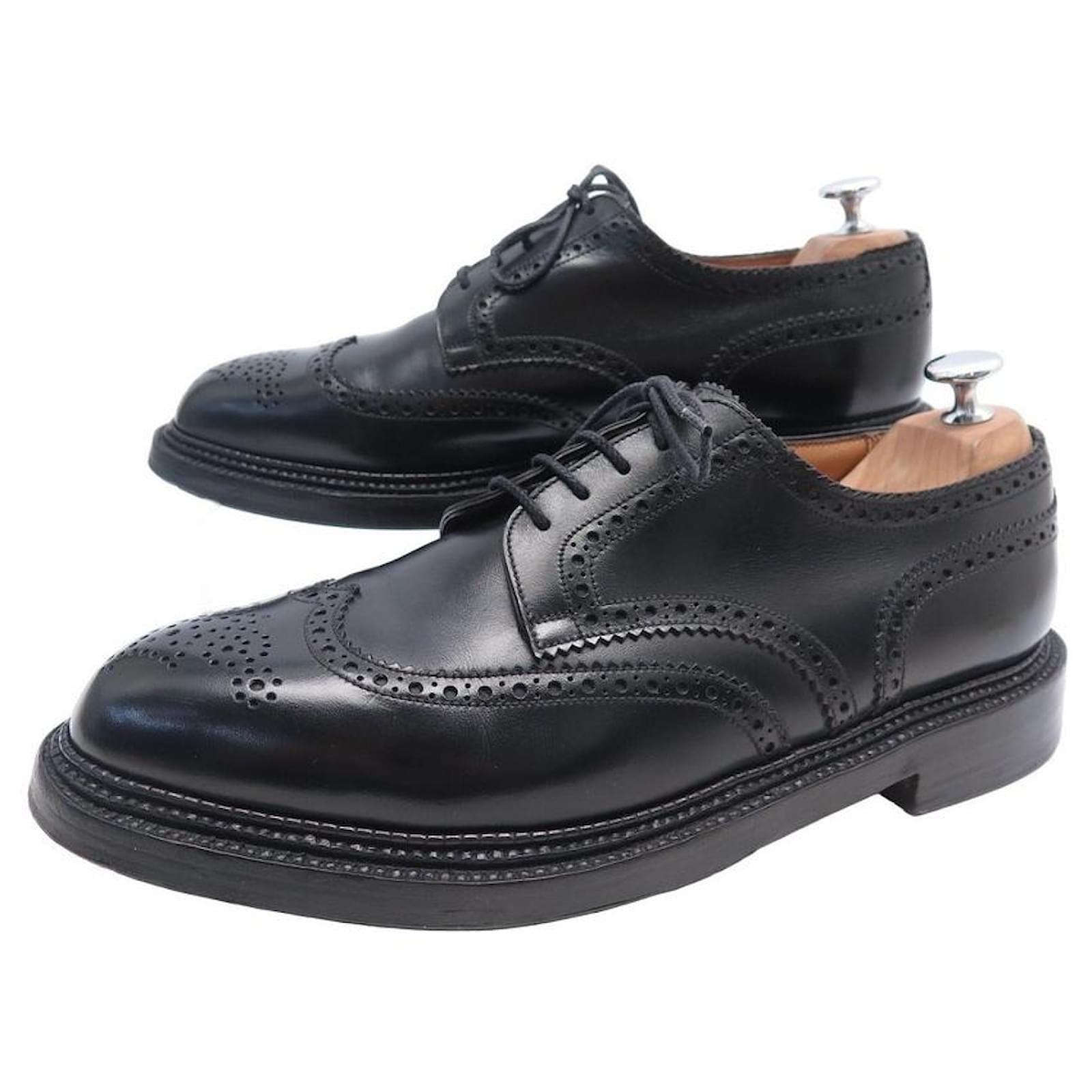This photograph depicts a pristine pair of men's black leather Oxford wingtip dress shoes resting on a white background. The shoes are characterized by their impeccable shine and neatly tied thin black laces. They feature a distinct pattern of small semi-circle decorative holes along the toe and consistent throughout the design, including on the laces. The shoes have a very low, small heel and triple-edged threading around each side. Inside each shoe is a wooden shoe horn, equipped with silver handles, intended to maintain the shoes' shape over time. The soles exhibit a solid black color, indicating that the shoes are not worn down at all.